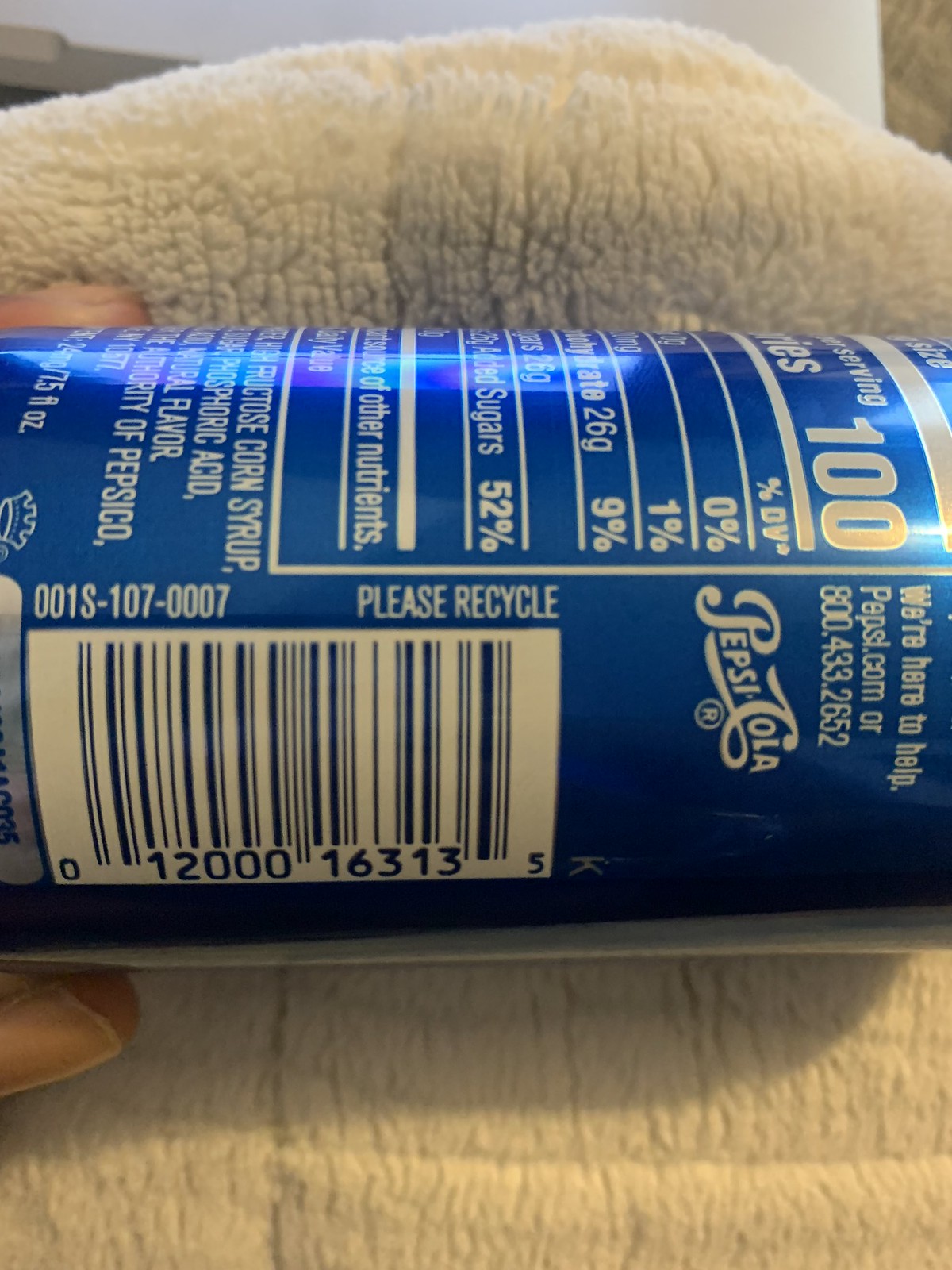This detailed photograph showcases a horizontally positioned blue Pepsi Cola can, prominently displaying the back and side views. At the top of the can, the nutritional information is partly visible, highlighting "100 calories" and various sugar and carbohydrate percentages. The right side of the can features the "Pepsi Cola" logo, while the top right corner includes the text, "We're here to help: pepsi.com or 800-433-2652." A barcode with the sequence "1-2-0-0-0-1-6-3-1-3," along with a "please recycle" message, is located toward the bottom left. The can rests on a beige, fluffy fabric, and a person's fingers delicately hold the bottom left of the can, their hand partially visible in the image.